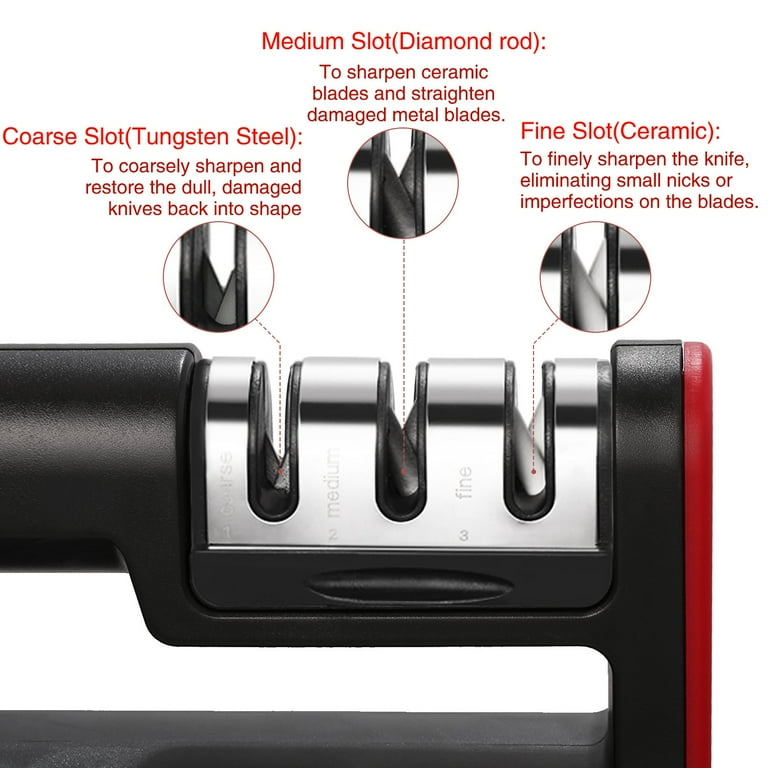The image is a close-up photograph of a robust, well-made knife sharpener, predominantly black with a distinctive red rim and handle. This precision instrument features a rectangular metal section with three distinct sharpening slots. Each of these slots is detailed with red text, providing specific instructions and descriptions. The leftmost slot, labeled "Coarse," uses tungsten steel to coarsely sharpen and restore dull or damaged knives. The middle slot is marked "Medium" and utilizes a diamond rod to sharpen ceramic blades and straighten damaged metal blades. The rightmost slot, labeled "Fine," is ceramic and designed to finely sharpen knives, eliminating small nicks and imperfections. Additionally, the image includes magnified views of each slot, highlighting their unique structures and purposes, making it evident that this knife sharpener is engineered to address various levels of blade wear and precision.